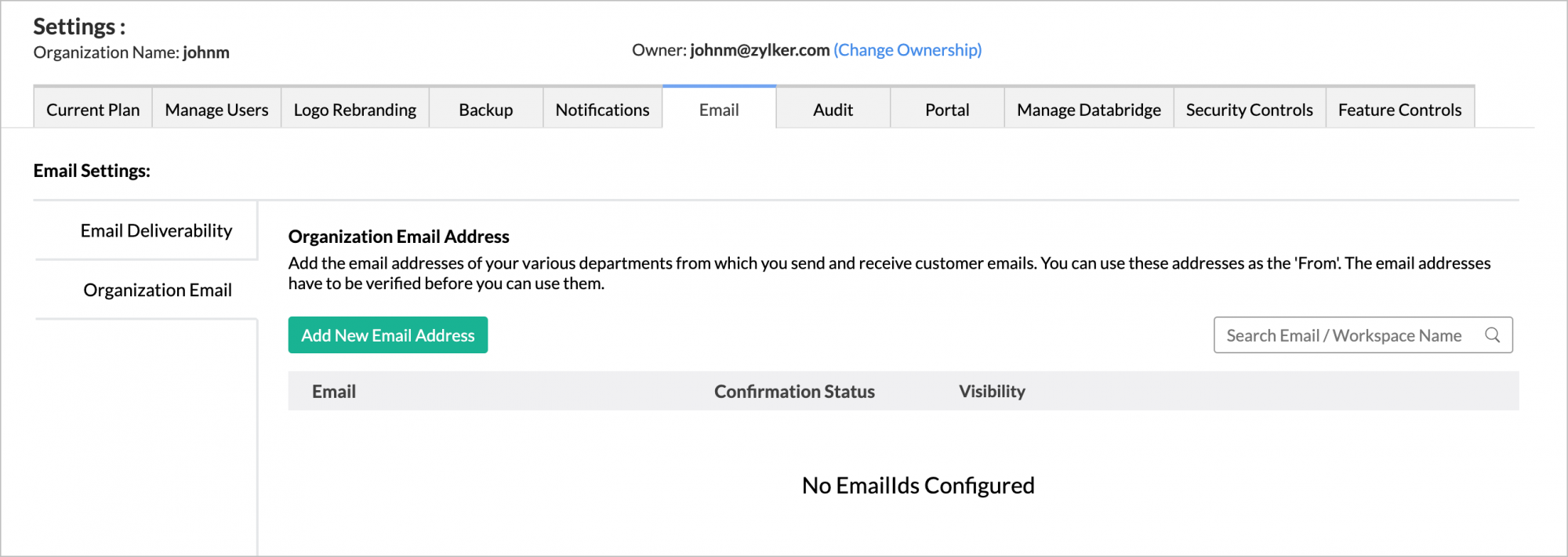The image depicts a screenshot of an application window displaying the settings menu. In the upper left corner, black text indicates the hierarchical navigation as "Settings: Organization Name: John M." At the top center of the image, the text "Owner: John M at zilcar.com" is prominently displayed, accompanied by a blue link labeled "Change Ownership." Below the header, a variety of settings options are laid out horizontally from left to right, including: "Current Plan," "Manage Users," "Logo Rebranding," "Backup," "Notifications," "Email" (which is highlighted), "Audit," "Portal," "Manage Data Bridge," "Security Controls," and "Feature Controls." The left side of the image features a vertical menu specifically for "Email Settings."